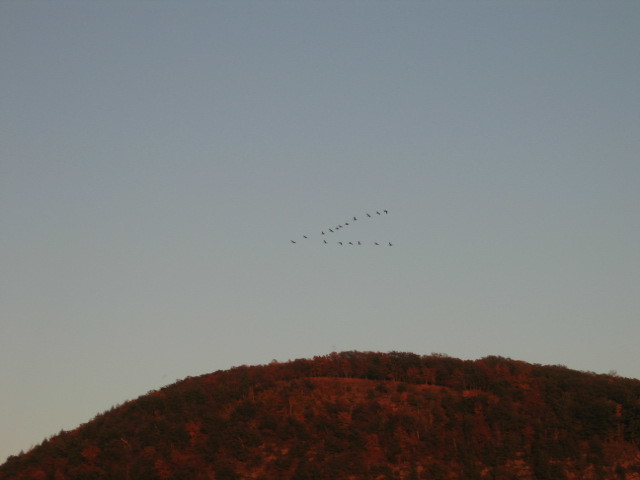The photograph captures a gently curved hillside or small mountain during either the autumn season or sunset. The hillside prominently features reddish-brown colors interspersed with scruffy, dense trees and a sizeable bare patch towards the top middle. In the background, a slightly hazy sky transitions from light blue to a subtle yellow gradient, suggesting the approach of dusk or the influence of a setting sun. Fleeting across the center of the image is a distant flock of around 17 birds, arranged in a V-formation. These black silhouettes are meticulously flying towards the left-hand direction of the photo, appearing as tiny dots against the expansive sky. With no visible buildings and the natural elements taking center stage, the scene conveys a tranquil and unspoiled landscape.